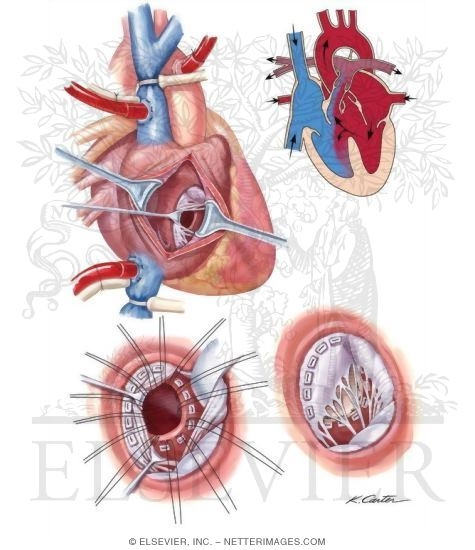This is a medical textbook illustration of the human heart, displaying four detailed views in color. The primary image in the top left shows the heart being operated on with metal tools and clamps pulling open the tissue. The top right illustration presents a flat diagram of the heart with red and blue arrows indicating blood flow through the various valves. The right side, colored red, represents oxygenated blood being pumped out, while the left side, colored blue, depicts deoxygenated blood flowing into the heart. The bottom images appear to be close-ups of specific regions of the heart shown in the top illustrations. These close-ups highlight the internal structures and membranes, with tools widening openings and strands visible within the cavities. Throughout the image, color coding is used to differentiate between various anatomical elements, with the heart itself in a pinkish hue, and some parts highlighted in blue or red. The illustration has a copyright notice from Elsevier Inc. and Netterimages.com, as well as an unreadable signature in the bottom right corner.